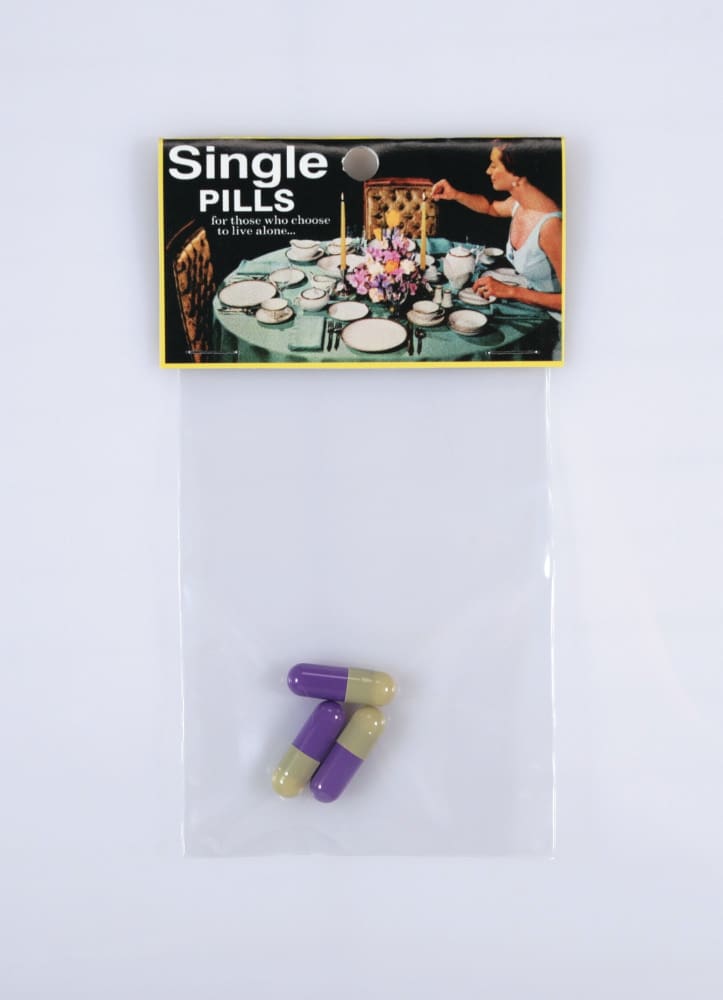This image features a package of "Single Pills," a product seemingly designed as a satire intended for those who choose to live alone. The package consists of a clear plastic bag pinned to a wall against a grayish background. The top of the package has a black label with the text "Single Pills" in white letters. Just below the label, there's an illustration that adds to the humorous theme: a woman with dark hair, wearing earrings and a light-colored dress, is seen sitting alone at a finely set, round table. The table is adorned with a plate, teacup, saucer, salad plate, utensils, and a light green linen napkin, with four place settings in total. At the center of the table, there are two long candles and a floral arrangement consisting of purple and white flowers. The woman in the picture is depicted lighting one of the candles. Directly below this image, the clear plastic bag contains three purple and beige capsule pills. The scene is likely intended for a humorous or satirical context, perhaps as a gag gift among friends. The colors in the image include gray, white, black, brown, red, blue, purple, and off-white.